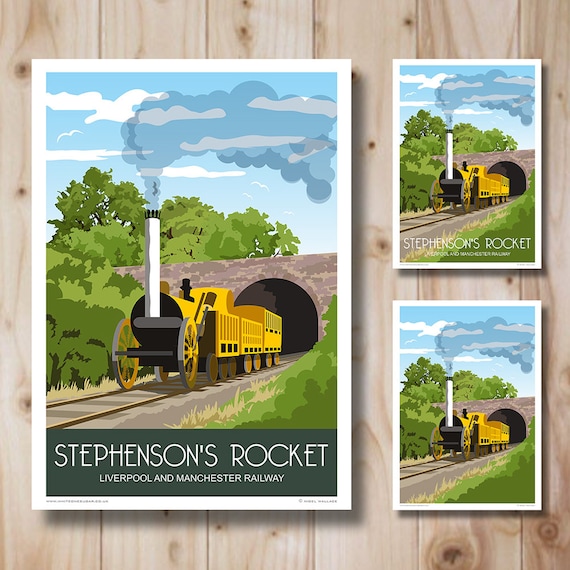In this square image, three posters are arranged against a light wooden surface with vertical slats and dark knots. The large vertical rectangular poster on the left is framed with a white border. The two smaller posters to its right are identical in image, depicting a yellow steam engine with brown circular wheels emerging from a stone tunnel. The tunnel is topped by a stone bridge with green trees and bushes around it. The steam engine emits gray smoke into a blue and white sky. The large poster on the left features text at the bottom: "Stevenson's Rocket, Liverpool and Manchester Railway." The top smaller poster also includes the text "Stevenson's Rocket" but omits the additional railway line, while the bottom smaller poster has no text. This scene is presented either on a wooden wall or lying flat on a wooden floor.